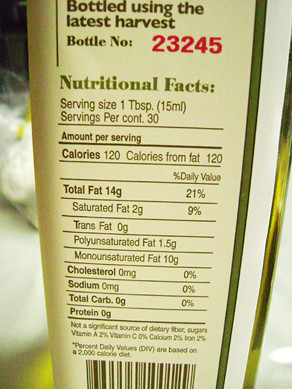A close-up image showcases the side panel of a packaging box, with its white background and green text prominently displayed. The box rests on a counter or table, with a slightly blurred background visible to the left, adding depth to the composition. A subtle greenish glow at the bottom creates a visually appealing effect. The text on the box states "Bottled using the latest harvest, bottle number 23245," with the bottle number emphasized in bold red. The nutritional facts are also clear: serving size of one tablespoon, 30 servings per container, 120 calories per serving, all from fat totaling 14 grams. A black UPC code is situated at the bottom, while a green vertical stripe accentuates the edge of the box, lending a clean and straightforward appearance. This intimate, detailed photograph appears to be taken with the purpose of conveying specific product information.